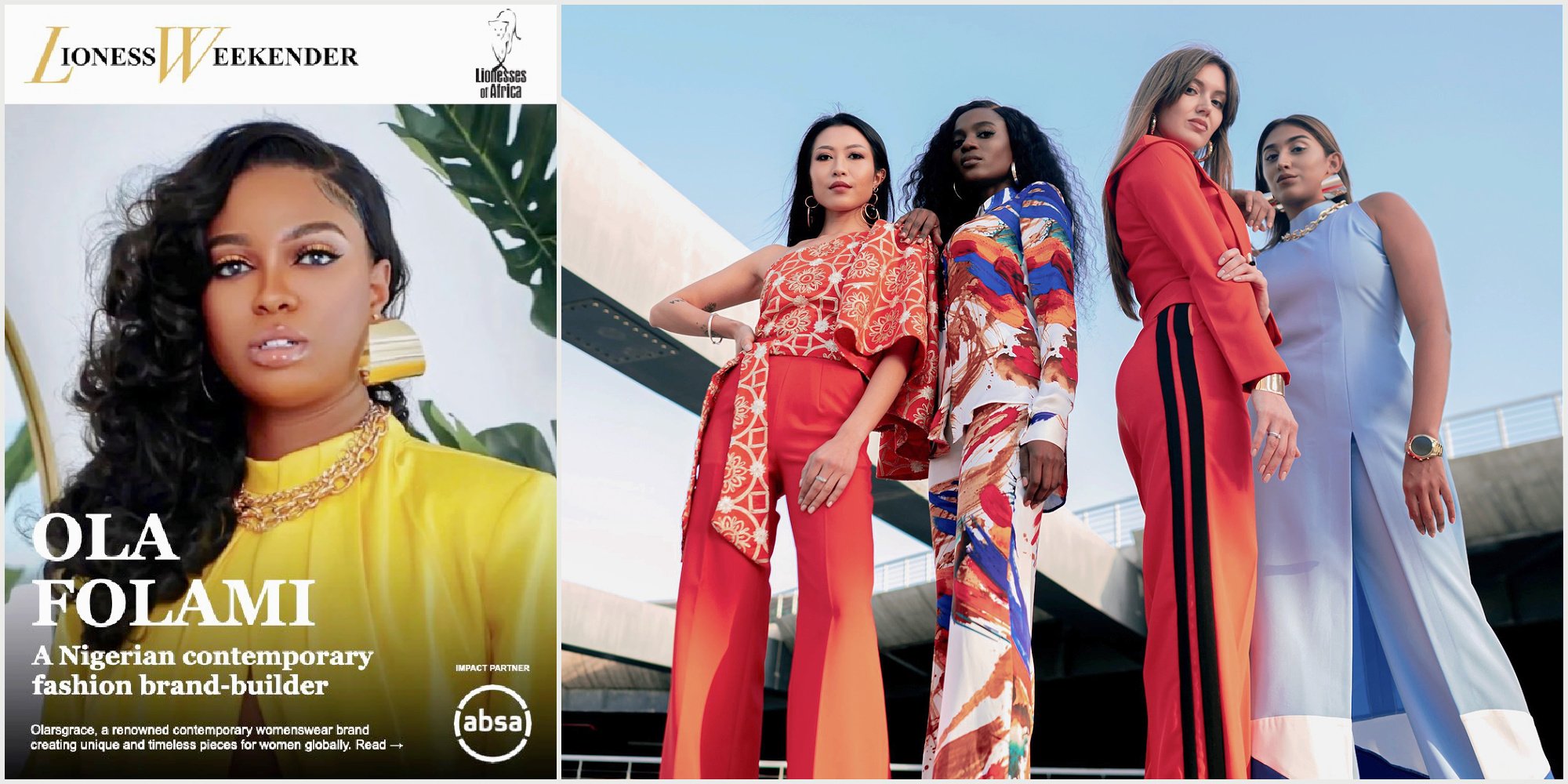The magazine cover of "Lioness Weekender," an African publication, prominently features a striking image of a black woman with elegant makeup, adorned with large gold earrings, a cascading mane of black curls over her right shoulder, and a gold necklace. She is wearing a vibrant yellow shirt. The text identifies her as Ola Folami, a renowned Nigerian contemporary women’s wear brand builder. The cover highlights her fashion accomplishments and includes a mention of "Lionesses of Africa," and their partnerships with ABSA. Adjacent to her image, an advertisement showcases four diverse models standing, viewed from a low angle that emphasizes their full body lengths. They are donning an array of brightly colored outfits: the first model in reddish-orange pants and a patterned shirt, the second in a multicolored jumpsuit combining blue, orange, and white hues, the third in a red tracksuit with black stripes, and the fourth in a blue ensemble that could be either a dress or a romper. Each model’s attire reflects the vibrant, contemporary fashion of Ola Folami’s brand.